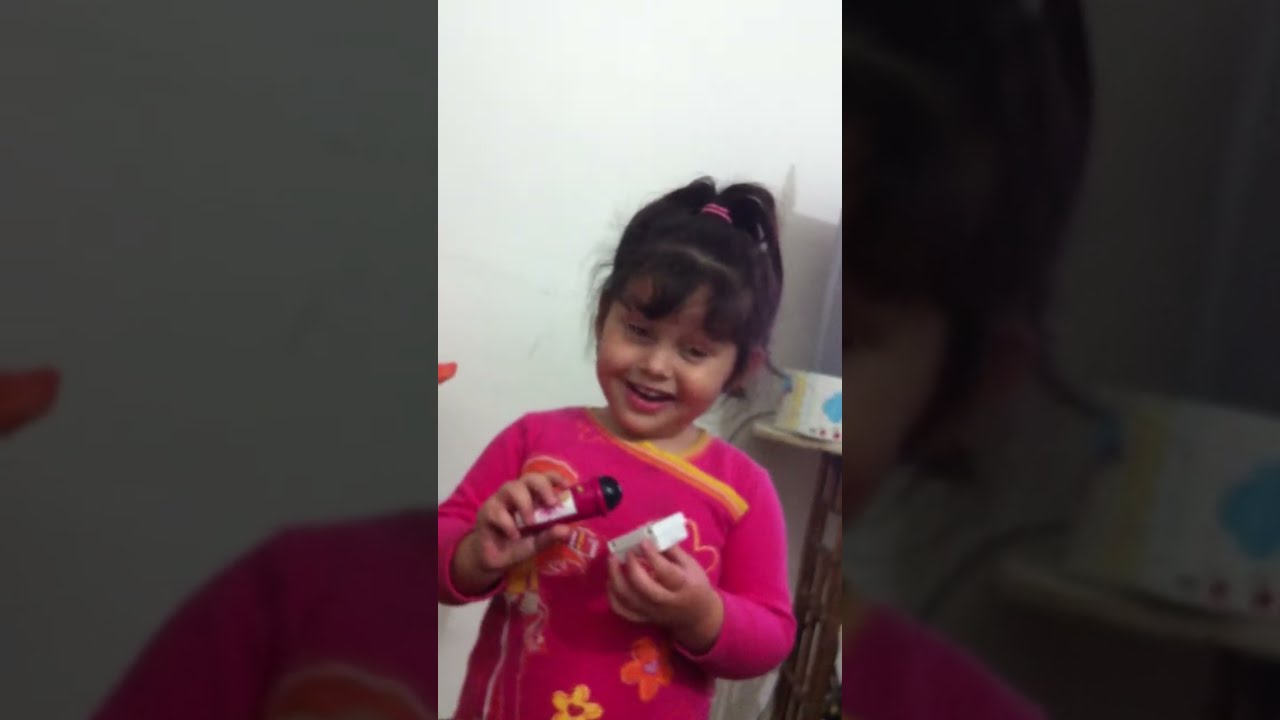In this color photograph, presented in portrait orientation, a young girl stands smiling in the center of the image. She has dark hair pulled back into a ponytail with a pink scrunchie. She wears a bright pink long-sleeved shirt adorned with yellow around the collar and decorated with yellow and orange flowers, as well as other small doodles partially obscured by her hands. The girl is holding two objects: a small white rectangular box in her left hand and a red bottle with a black cap in her right. Though she is smiling, she is looking slightly towards the bottom of the camera rather than directly at it. The background features a blank white wall, a small table on her right with what appears to be a tissue box, and an orange stand partially visible on her left. The setting appears to be indoors, possibly in a living room or a child’s bedroom, and no text is present in the image. The overall style of the photograph is photographic representationalism realism.